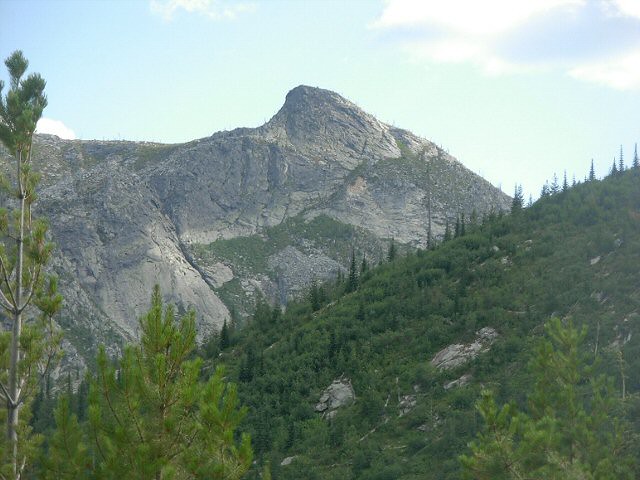The image is a rectangular photograph depicting a picturesque outdoor scene of a mountainside. The sky is a light blue, scattered with fluffy white clouds, particularly concentrated in the upper right-hand corner, which partially obscure the bright sunlight. Most prominently in the background, a large, rocky summit dominates the view, its gray stone surface interspersed with sparse greenery clinging to its sides. This majestic peak, devoid of trees and appearing rugged with jagged rocks, seems to be far off in the distance.

In the foreground, a smaller, rolling hillside covered in lush, green vegetation, primarily evergreen and fir trees, unfolds from the lower left-hand side of the image, ascending diagonally towards the middle right. A narrow tree trunk, likely a pine tree, with its leaves partly visible, adds to the scene's verdant charm. There is no sign of animal or human presence, no birds in the sky, nor people or vehicles; the scene is tranquil and undisturbed, capturing the serene beauty of nature.